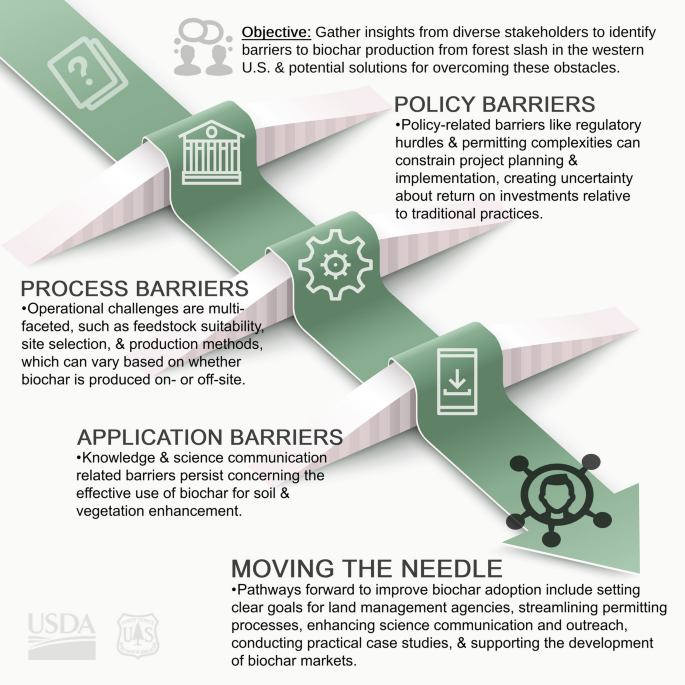The image is an educational poster issued by the USDA, designed in olive green and white. It revolves around the objective of gathering insights from diverse stakeholders to identify barriers to biochar production from forest slash in the Western U.S. and to propose potential solutions for overcoming these obstacles. At the top, the poster prominently states the objective. A central green stripe, transitioning into an arrow, visually symbolizes progress by traversing various barriers and pointing downwards. On the right side, it details policy barriers such as regulatory hurdles and permitting complexities, which can hinder project planning and create uncertainty about returns on investments compared to traditional practices. To the left, it addresses process barriers like feedstock suitability, site selection, and production methods. Below, it elaborates on application barriers, emphasizing challenges in knowledge and scientific communication that affect the effective use of biochar for soil and vegetation enhancement. The bottom section, titled "Moving the Needle," looks ahead to potential future adaptations. Various symbols, including cards, a house, a ship, a gear, and an arrow, are interspersed among the text, with USDA and U.S. symbols at the bottom, setting the context for this comprehensive overview.